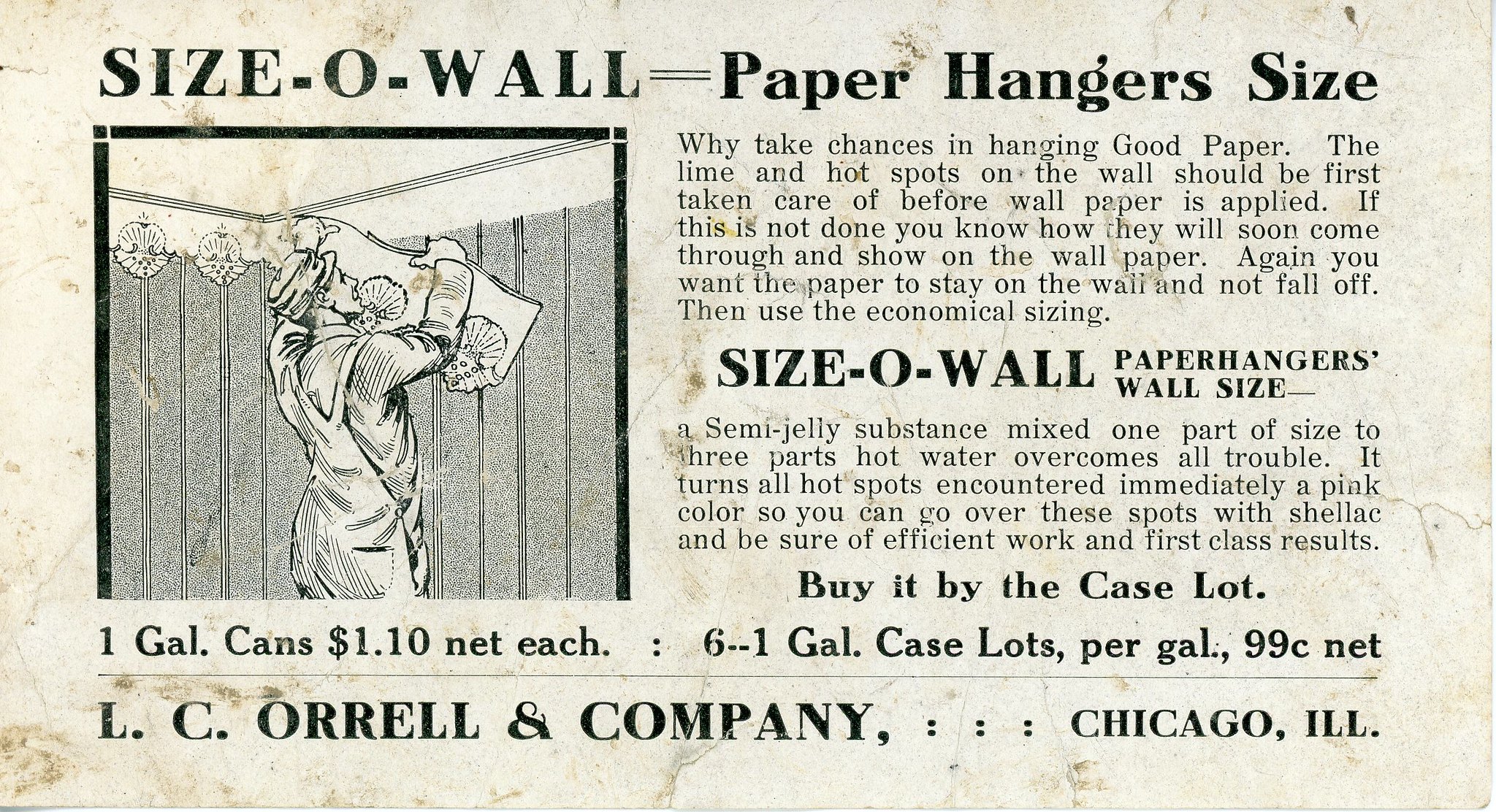This rectangular, black-and-white image appears to be an aged label or excerpt from a newspaper, showing signs of yellowing with time. Dominated by text, it features a small illustration on the left side of a man in work overalls meticulously hanging wallpaper. The prominent headline across the top reads: "Size O Wall = Paper Hanger Size." 

The accompanying article advises on the proper preparation for hanging wallpaper, emphasizing the importance of addressing imperfections on the wall before application. The text explains that untreated lime and hot spots can damage the wallpaper if not fixed beforehand. To ensure the wallpaper adheres properly and stays intact, it recommends using an economical sizing solution called "Size O Wall Paper Hangers Wall Size." This solution, described as a semi-jelly substance, should be mixed in a ratio of one part size to three parts hot water. The mixture instantly turns hot spots pink, allowing for precise application of shellac to secure a flawless finish.

The product is sold by the case, priced at $1.10 per one-gallon can, with a discount lowering the price to $0.99 per gallon when purchasing six one-gallon case lots. The bottom of the image is marked with the manufacturer's details: "L.C. R.L. and Company, Chicago, Illinois."